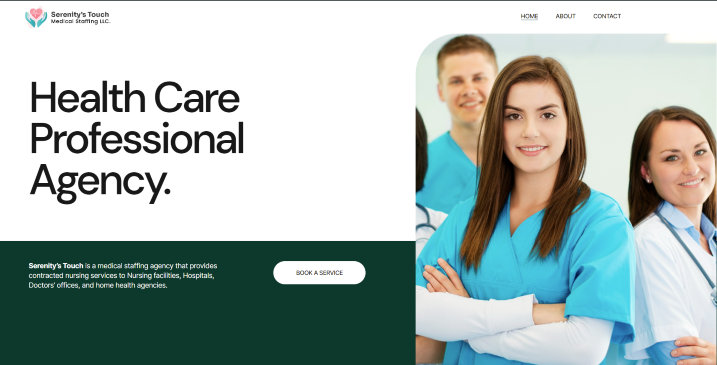A website screenshot showcasing Serenity's Touch, a medical staffing agency. The top left corner features the logo 'Serenity's Touch' with smaller text beneath it mentioning their medical staffing services. In the top right corner, navigational links for 'Home,' 'About,' and 'Contact' are presented in black text against a white background. The main headline on the left reads 'Healthcare Professional Agency.' To the right of the headline, there is a photo depicting several individuals in medical attire. 

At the forefront, a young woman, likely in her early 20s, stands confidently in a nurse outfit consisting of a green top with white sleeves underneath, suggesting she has recently completed nursing school. Beside her, another woman dressed in a white shirt appears to be a medical assistant or possibly a junior medical professional. Behind them, a male nurse is also visible in the same green top uniform. 

Below the headline, text introduces Serenity's Touch as a medical staffing agency that provides contracted nursing services to various healthcare facilities, including nursing homes, hospitals, doctor's offices, and home health agencies.